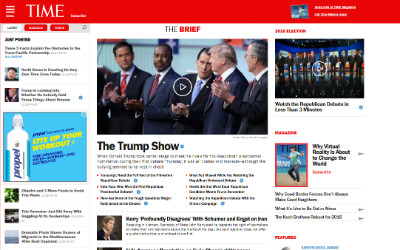This is a detailed descriptive caption:

"A screenshot of the Time Magazine website, displayed with very poor resolution, making most text unreadable. The characteristic red bar at the top features the 'Time' logo in white. Below it, the section titled 'The Brief' stands out, with 'The' in black and 'Brief' in red. To the right, a headline related to an election is partially visible in red. Dominating the page is a blurred image of Donald Trump surrounded by his supportive Republicans, referred to as 'The Trump Show' in black text beneath the image. Adjacent to the main story are thumbnails of additional articles, one concerning Trump with an image of Kim Jong-un and another related to cars. The entire web page suffers from severe resolution errors, making finer details and navigation buttons impossible to discern. The main feature includes a play button overlay on the picture, suggesting a video related to 'The Trump Show.'"